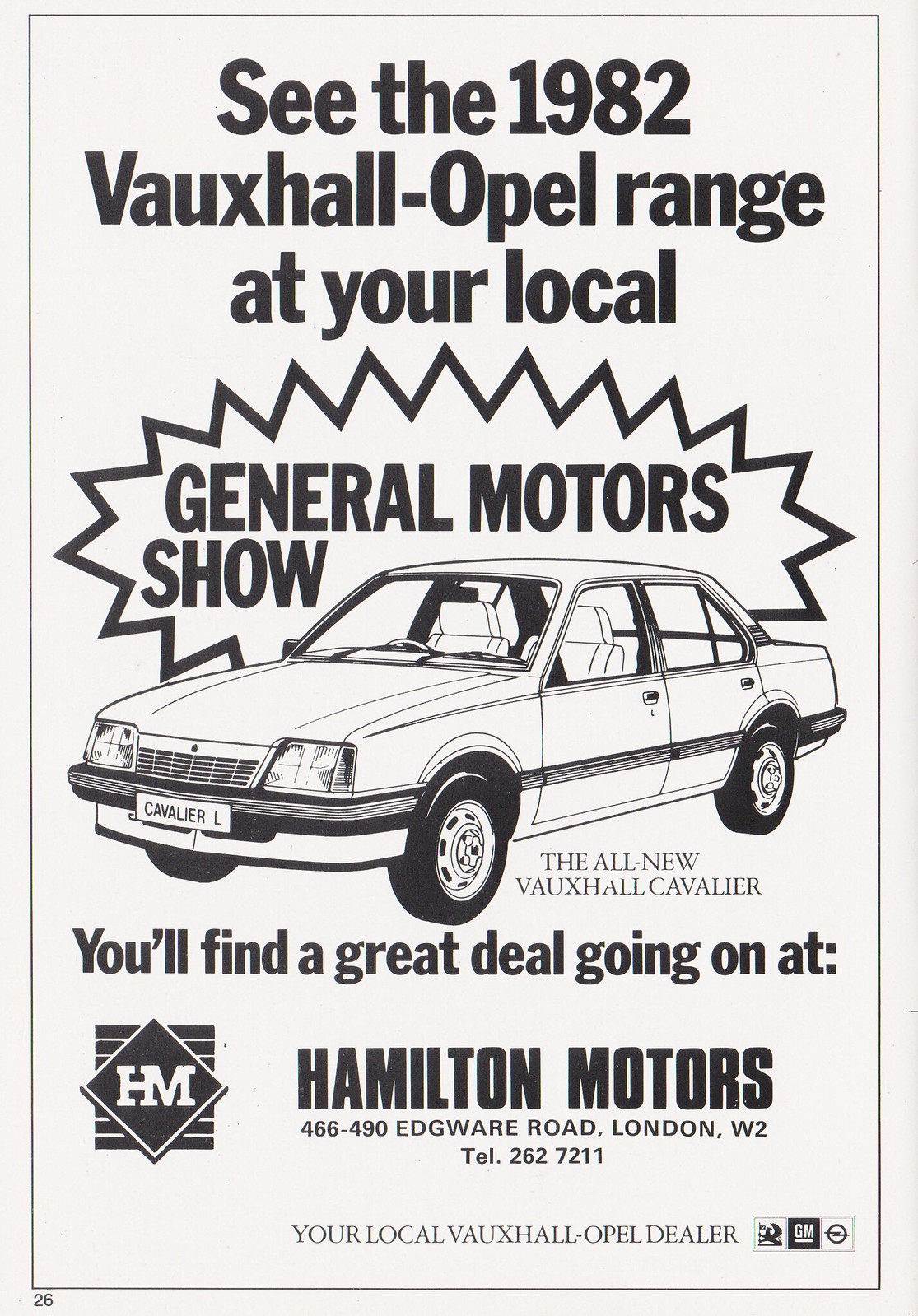This black and white advertisement showcases the 1982 Vauxhall Opel range, prominently featuring the all-new Vauxhall Cavalier L. At the center, an illustrated four-door model displays its Cavalier L plate, emphasizing the car's new introduction. The top of the ad invites viewers to "see the 1982 Vauxhall Opel range at your local General Motors show." Below the car's illustration, bold text promises, "you'll find a great deal going on at Hamilton Motors," with the address, "466-490 Edgeware Road, London, W2" and a telephone number "262 7211". The bottom of the image also identifies Hamilton Motors as "your local Vauxhall Opel dealer." A GM logo is positioned to the left of the dealership details. The ad, with its stark black and white design, reminiscent of newspaper clippings or old posters, distinctly reflects a bygone era of car advertisement.